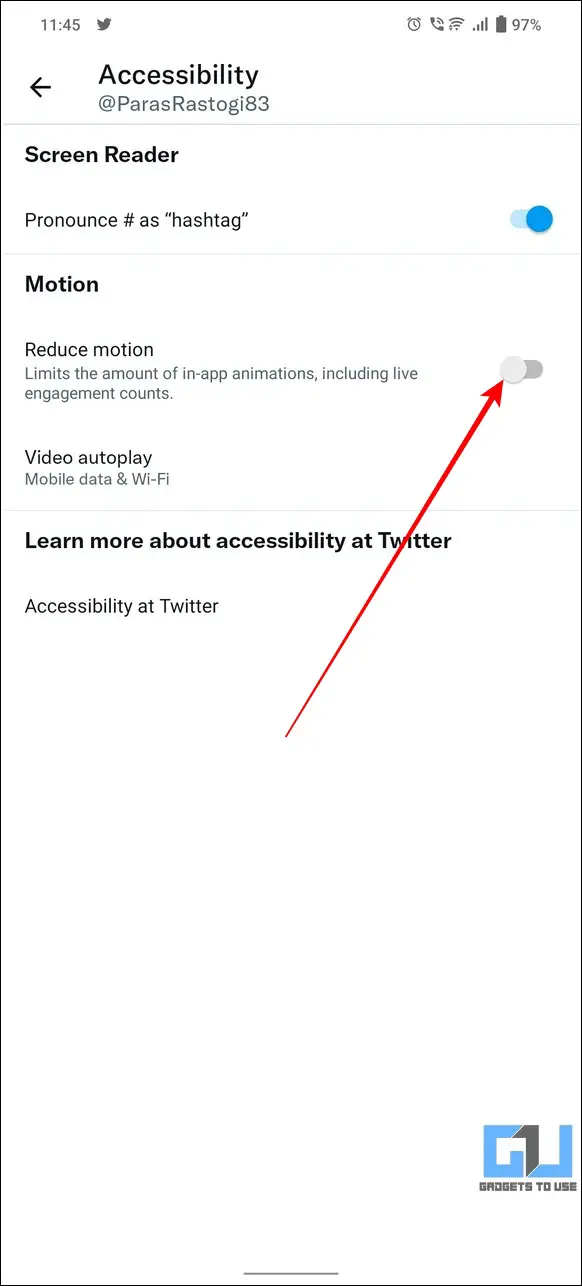The image is a screenshot of a vertical webpage with a thin black border against an all-white background.

At the very top, the digital clock displays the time as 11:45. To the right of the time, there is the Twitter bird logo, followed by icons for an alarm clock, a ringing phone with curved lines indicating sound, a Wi-Fi signal, a cell signal, and a battery icon showing 97% charged.

Beneath the icons, there is a back arrow on the left side, rendered in black, and next to it, an accessibility icon represented by a capital "A". Below this, the username "@ParasRastogi83" is prominently displayed, with 'Paras' and 'Rastogi' capitalized, indicating a Twitter profile handle.

The next section features a screen reader setting that states "Pronounce the pound sign as 'hashtag'", with "hashtag" enclosed in quotation marks. This setting is shown as enabled.

Continuing down, there is a section labeled "Motion" in bold text. Below this header, there is an option reading "Reduce motion", which concerns the amount of in-app animations, including live engagement counts. This setting is depicted as turned off, with a red arrow pointing to the off circle.

Further down, another option titled "Video autoplay" indicates settings for mobile data and Wi-Fi. At the bottom, there is a call to action in bold text that reads, "Learn more about accessibility at Twitter," followed by a plain text link, "Accessibility at Twitter."